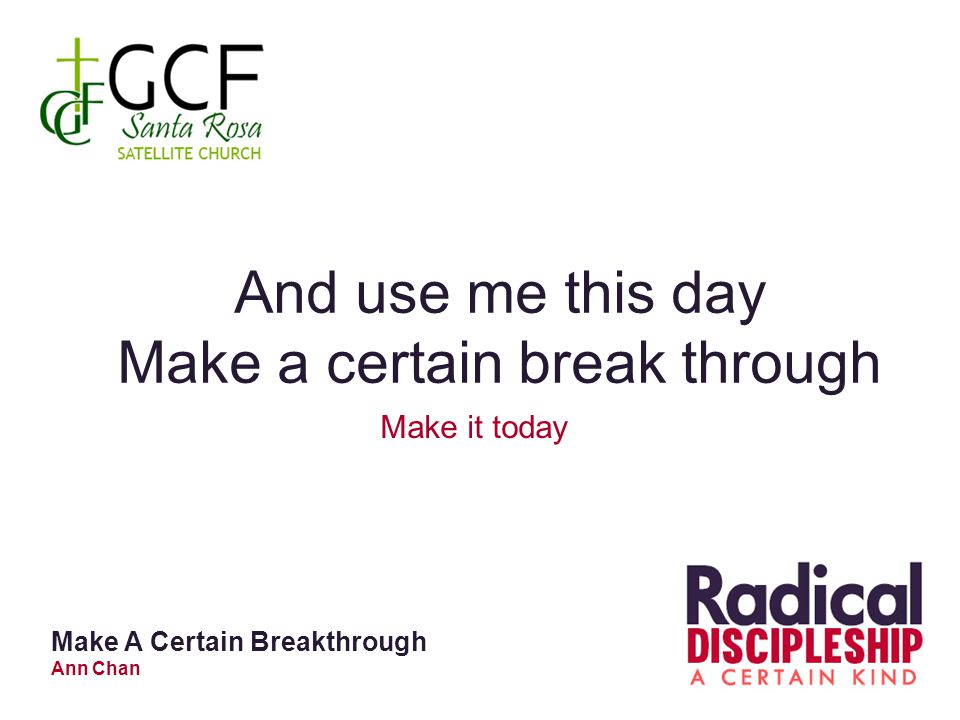The image features an informational sign or advertisement with a white background. At the top left, there's a logo of the GCF Santa Rosa Satellite Church, which includes a green cross intertwined with the darker green letters GCF. Just to the right of this logo, the text spells out "GCF Santa Rosa" in black and dark green, with "Satellite Church" in light green below it.

Centered in the image, the main title in black text reads: "And use me this day, make a certain breakthrough." Directly underneath this, in a smaller red font, is the phrase "Make it today." On the bottom left, the text again states "Make a certain breakthrough," this time as a single word in black font. Below this, in red font, is the name "Ann Chan."

On the bottom right of the image, the words "RADICAL" in grey and "DISCIPLESHIP" in red all caps are displayed, followed by "A CERTAIN KIND" in orange all caps, in a smaller font. The layout uses a variety of colors and font sizes to emphasize different parts of the message.